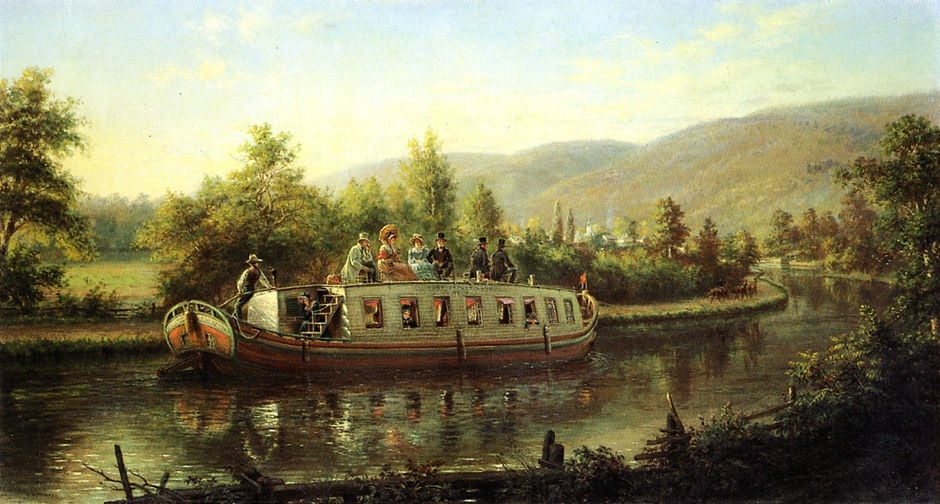This is a vintage oil painting from the early to mid-1800s, depicting a serene river scene featuring a houseboat or barge carrying wealthy Victorian-era tourists. The white and orange boat, adorned with shingles and cutout windows along the sides, is gliding down a peaceful, meandering river that eventually curves to the left. The boat has an enclosed level with windows, accessible by a small set of stairs leading to a viewing platform or roof. On the roof, six people—three men in black top hats and Victorian suits, and three women in brownish-orange and blue dresses—are enjoying the tranquil day. A driver stands at the back, steering the vessel. The backdrop is a picturesque landscape with low hills, trees lining the riverbanks, patches of grasses, sticks, and branches. Above, the sky is dotted with white clouds, and distant mountains complete the idyllic scenery. The muted colors enhance the peaceful and timeless quality of this bucolic scene.